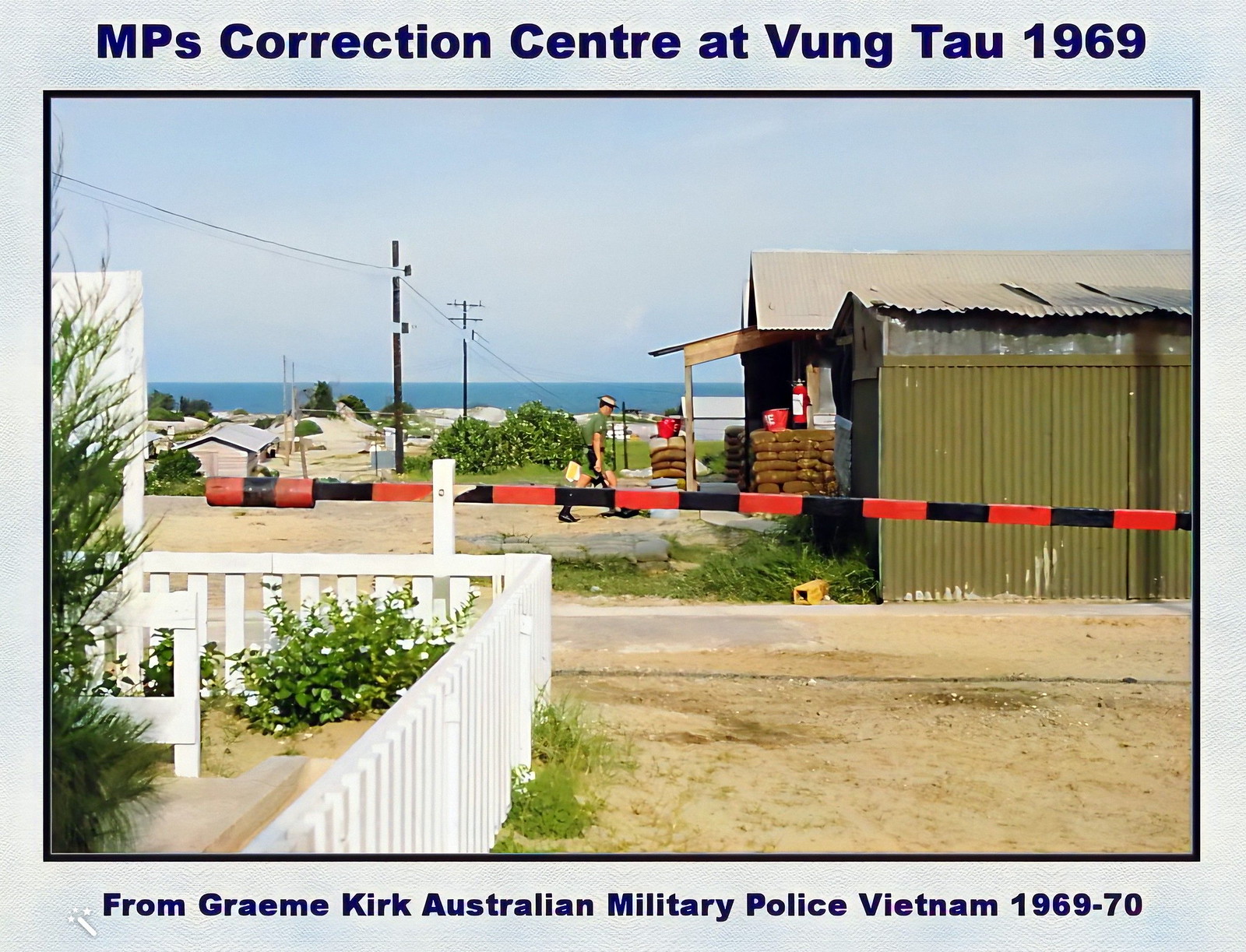The rectangular horizontal photograph with a light blue and white border and blue text at the top reading, "MPs Correction Center at Vung Tau, 1969," captures a military scene from the era of the Vietnam War. The text at the bottom identifies the source: "From Graeme Kirk, Australian Military Police, Vietnam, 1969-70."

Central to the image are several buildings, including a barrack with vertical green siding and a metal roof, and another structure featuring a brown porch and lighter roof. A uniformed soldier, clad in army green short-sleeve fatigues, green shorts, black socks, and boots, is seen walking toward the barracks, carrying a briefcase in his right hand. This soldier is set against the backdrop of telephone lines and white houses on the left, with blue water visible further in the distance under a clear sky.

In the foreground, stretching horizontally across the image is a black and red security gate, which bars vehicle entry. To the left of this gate, a white picket fence encloses an area with shrubs and flowers. A dirt road extends from the lower right up to the gate, with green grass and additional shrubbery adding to the scene’s detail and depth.